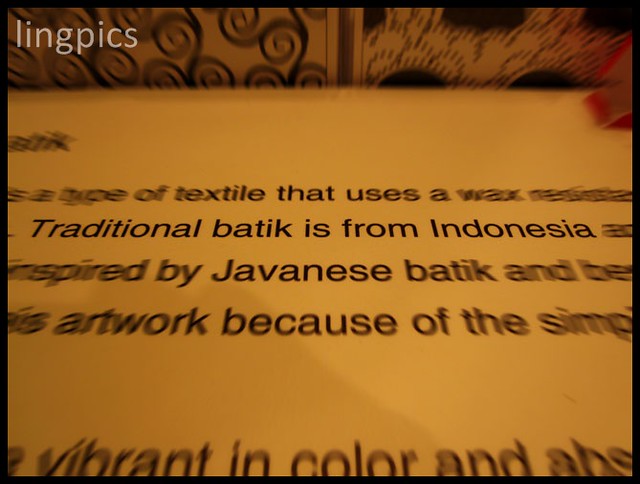The advertisement features the text "Lingpics" in light brown letters over a slightly darker brown background. It is framed by an elaborate border filled with curlicues and other line symbols, occupying about seven-eighths of the top portion of the image. The entire image is set within a thin, black rectangular border. A central section of the image contains various text elements, albeit somewhat difficult to read. Key phrases include "traditional batik is from Indonesia," and "type of textile that uses a wax," potentially indicating a focus on Javanese-inspired batik techniques. The overall aesthetic of the advertisement employs simple brown letters on a very light brown background, evoking a connection to traditional Indonesian batik art. Additionally, there is a watermark at the top that reads "Ling Pix" in light brown. The apparent purpose of the image is to describe the cultural and artistic heritage of batik textiles.